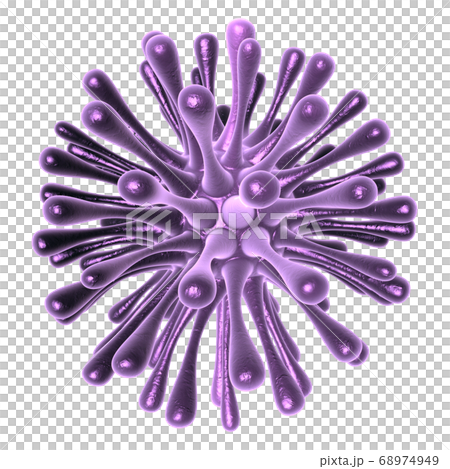The image features a computer-generated, purple starburst or splat-like figure with a dense, concentrated center and numerous curvy offshoots extending outward. These offshoots, numbering over 20 to 30, gradually darken from light purple at the center to black towards their ends, each finishing with a light purple point. The background is a small checkered pattern of gray and white squares, suggestive of a design that could disappear when integrated into documents, resembling a transparent background from clipart or paint programs. This complex form, somewhat reminiscent of a biological molecule or a collection of children's jacks, is digitally rendered and carries the text "Pixta.jp-68974949" in the bottom right-hand corner, indicating its source or creation style.